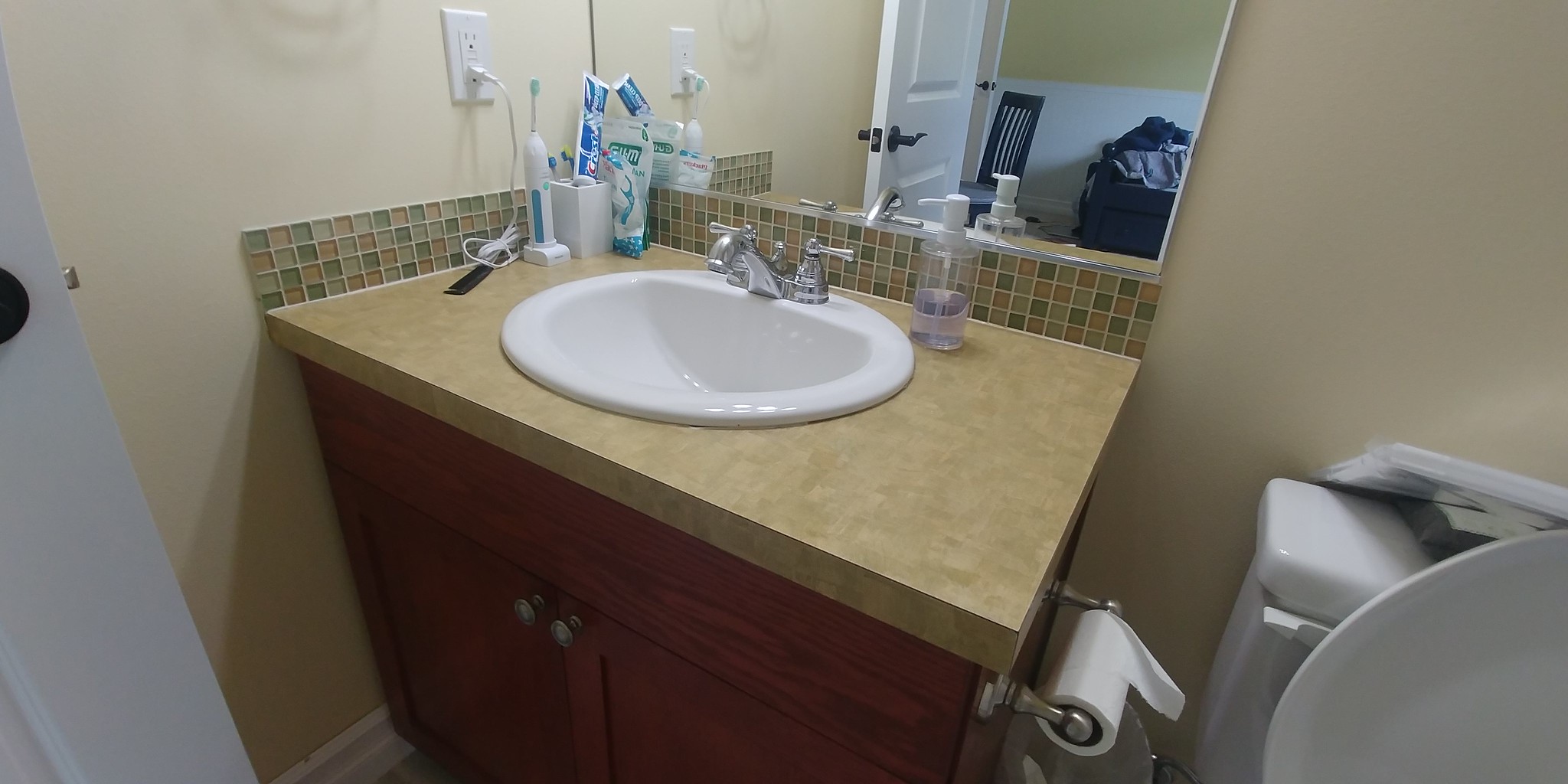This image depicts a compact, meticulously organized bathroom. On the left side of the frame, a partially open white door reveals the small space within. The central focus is a single vanity sink with a pristine white bowl and a gleaming silver faucet, equipped with separate handles for hot and cold water, positioned symmetrically on either side of the central spout. The vanity countertop, made of brownish granite, sits atop a cabinet of rich brown wood, adding a touch of elegance to the setting.

Adorning the walls around the vanity is a backsplash of mosaic tiles in a harmonious blend of neutral tones, including tan, brown, and hints of greenish-brown. Rising above the vanity is a standard mirror, exactly matching the width of the vanity, reflecting the hallway outside where a simple chair and a laundry hamper are visible.

To the left of the sink, an electrical outlet holds an Oral-B electric toothbrush, alongside various other dental care items. On the right side of the sink, a lavender-colored liquid soap dispenser stands ready for use. The right side of the vanity is also home to a toilet paper holder, presently bearing about a quarter-roll of toilet paper.

Partially visible to the right of the vanity is a white toilet, its lid open and the handle, like the rest of the fixture, starkly white. The overall aesthetic of the bathroom is clean, functional, and subtly stylish, with thoughtful details that create a welcoming and efficient space.